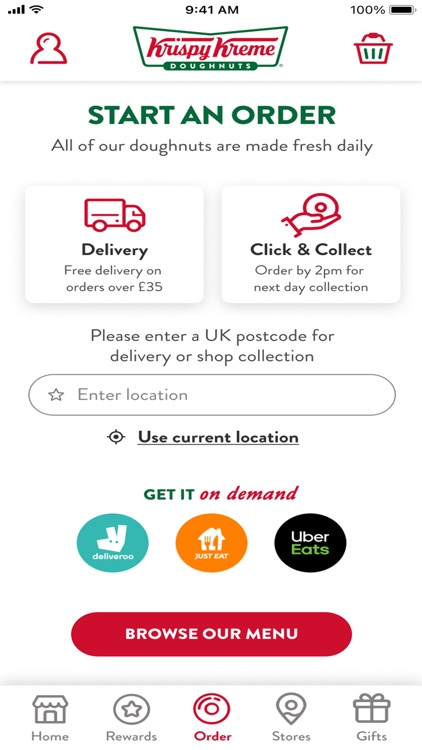**Detailed Caption:**

This is a detailed screenshot of the Krispy Kreme app interface taken from a cell phone at 9:41 AM, with the phone's battery fully charged at 100%. At the top center of the app, the Krispy Kreme logo is prominently displayed, featuring the trade name "Krispy Kreme" in bold red letters, underneath which "Donuts" is written within a bean-shaped word bubble background. To the left of the logo is an icon representing user accounts, and to the right, there's an icon that appears to be a trash can, though its exact function is unclear.

Below the header, the main body of the app starts with a prompt titled "Start an Order." It emphasizes that all donuts are made fresh daily. The interface provides two prominent buttons: one on the left labeled "Delivery" with an accompanying delivery truck icon, indicating this option is for delivering orders. The other button on the right is labeled "Click and Collect," detailing that orders placed by 2 PM will be ready for collection the next day, suitable for larger orders.

Further down, users are instructed to enter a UK postcode for delivery or shop collection in a provided text box, or they can opt to use the "Use Current Location" button to utilize GPS for automatic location detection.

Lower on the page is a section titled "Get it On Demand," featuring three buttons for various delivery services: Deliveroo, Just Eat, and Uber Eats, allowing users to choose their preferred platform for donut delivery. Beneath this is a big red button labeled "Browse Our Menu" for users to explore their options.

At the bottom of the app interface, there are navigational buttons labeled Home, Rewards, Order, Stores, and Gifts, providing easy access to different sections of the app.